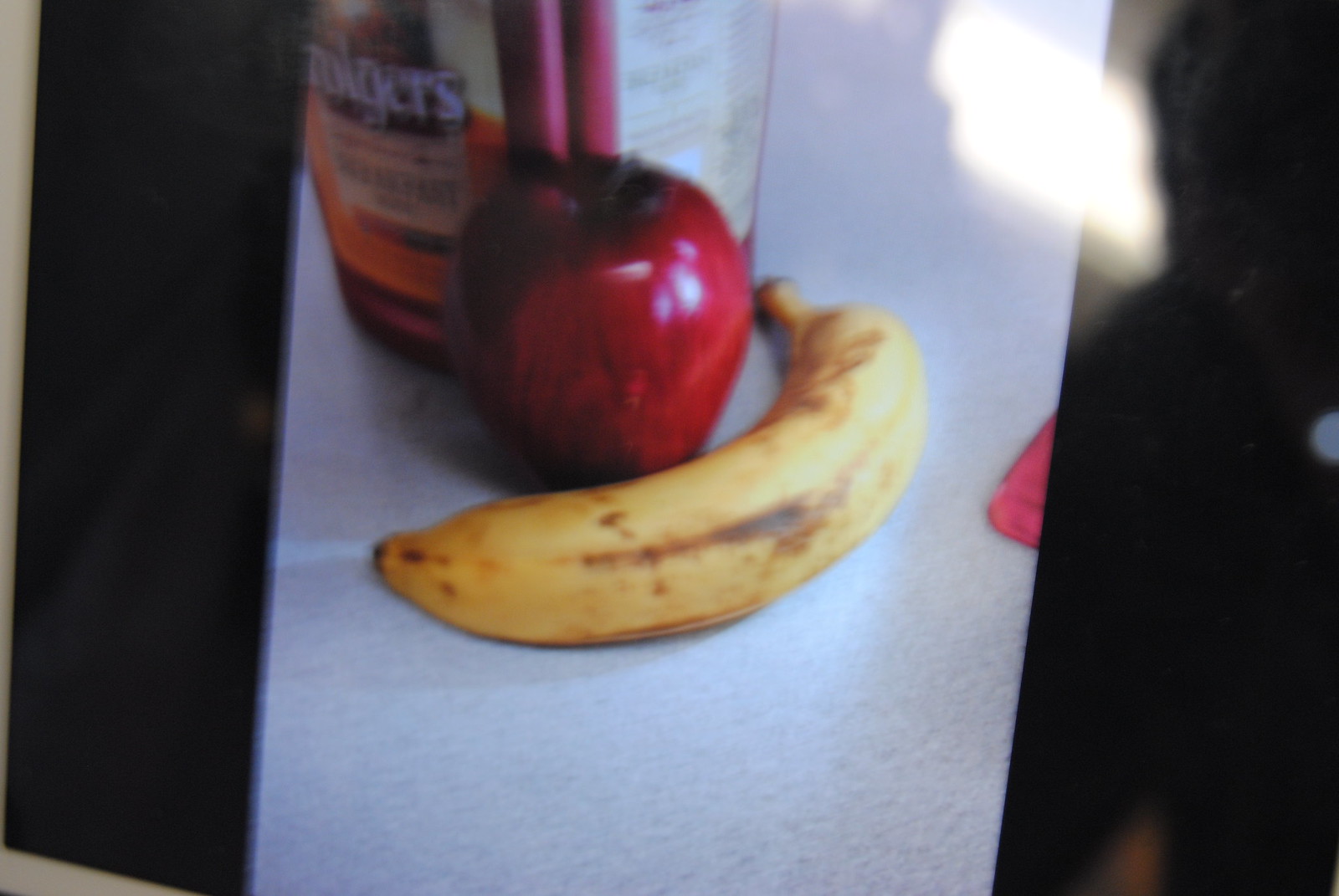The image depicts a digital display showcasing a photograph. The centerpiece of the photograph on the display is a ripe banana, identifiable by its browning spots. Positioned behind the banana is a red apple. Further to the rear, a red Folgers coffee can is visible, characterized by a beige and orange front label, although only "Folgers" is legible while the rest of the text remains blurry. The side of the canister also has a label, but its details are indistinct. The display screen exhibits black borders on both sides, creating the impression of a frame. In the upper right-hand corner, a light reflection reveals that this is a photograph of the screen. The left edge and bottom left corner show the white border of the device displaying the image. Additionally, there is a faint, unclear reflection on the right side, possibly of the individual taking the photo.